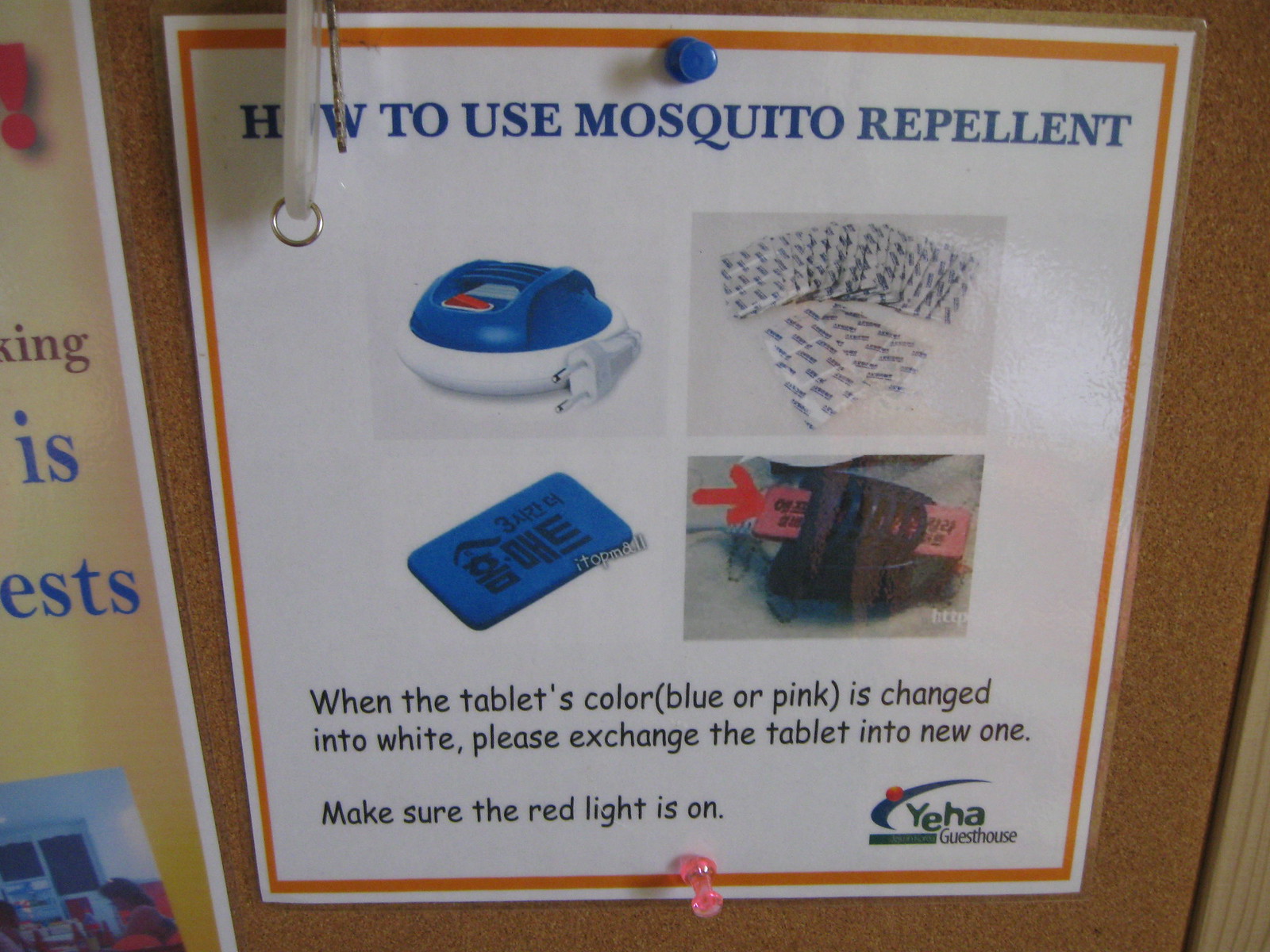The image depicts a detailed instructional poster for using a mosquito repellent device, affixed to a wooden brown door with colorful thumbtacks—a blue one at the top and a pink one at the bottom. The poster, primarily white with an orange border, bears the title "HOW TO USE MOSQUITO REPELLENT" in prominent blue capital letters. Centrally featured are four pictorial instructions: the top left shows the blue and white plug-in mosquito repellent device, the top right displays packets containing mosquito repellent tablets, the bottom left illustrates a single blue tablet (which can also be pink), and the bottom right demonstrates how to insert the tablet into the device, indicated by a red arrow. Below the images, black text instructs users: "When the tablet's color (blue or pink) changes to white, please exchange the tablet for a new one. Make sure the red light is on." Additionally, the bottom right corner of the poster houses the Yeha Guesthouse logo. To the poster's left, a partially visible adjacent poster with a yellow background and dark text is also noted.